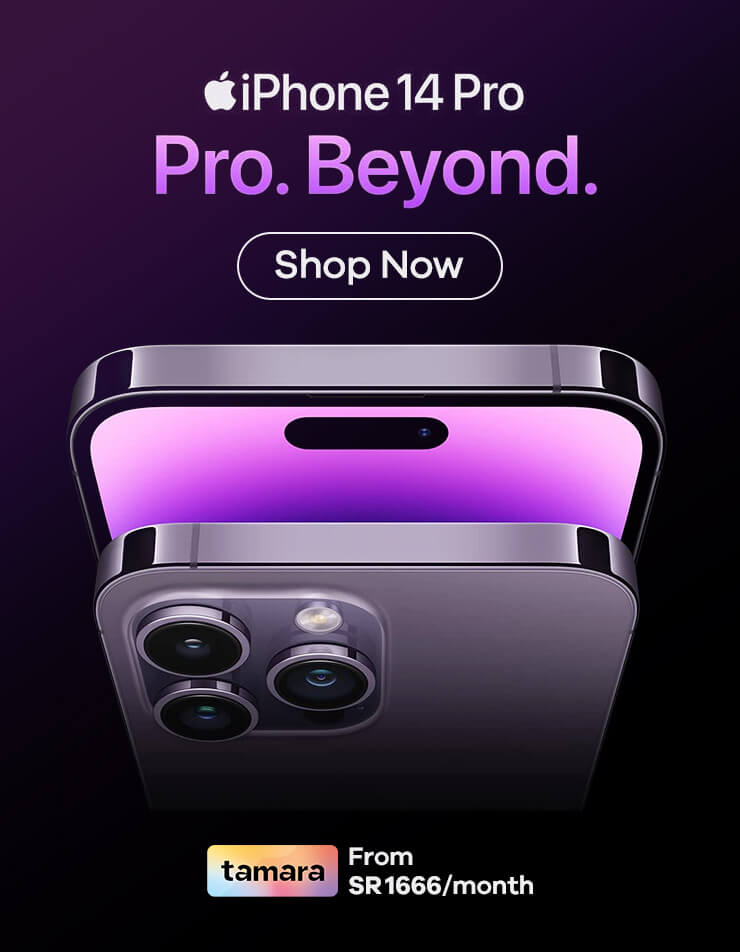A promotional advertisement for the iPhone 14 Pro showcases a sleek, animated graphic of the device, prominently featuring its distinctive three-camera setup on the pink-toned rear. The text "ProBeyond" appears in a bold pink font, emphasizing the advanced features of the phone. Above, the words "iPhone 14 Pro" are displayed in clean white lettering. The advertisement encourages viewers to "Shop Now" and notes that pricing starts at $16.66 per month. The overall design of the ad is modern and eye-catching, designed to appeal to those interested in the latest tech advancements.